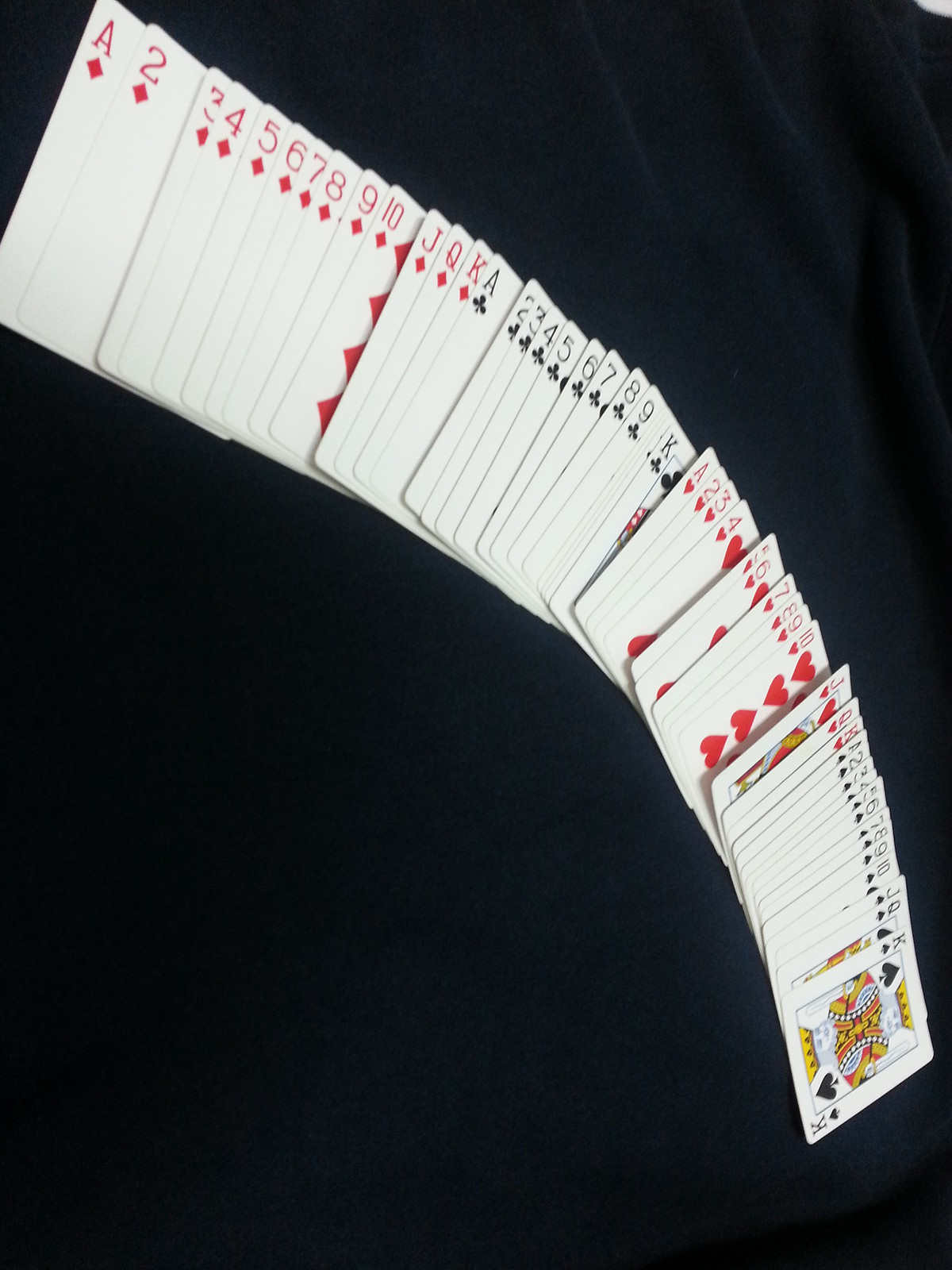A meticulously arranged collection of playing cards is spread out in a sequential order on a dark blue fabric backdrop. The cards are laid out in a neat arrangement, displaying the entire suit of Diamonds from the Ace to the King, followed by the Ace, Two, through to the King of Spades, the Ace through the King of Hearts, and finally, the Ace through the King of Clubs. Each card features a classic design with a white background and standard face values. The setting appears to be indoors, providing a focused, clean, and orderly presentation of the playing cards against the rich blue fabric, enhancing their vibrant colors and intricate details.